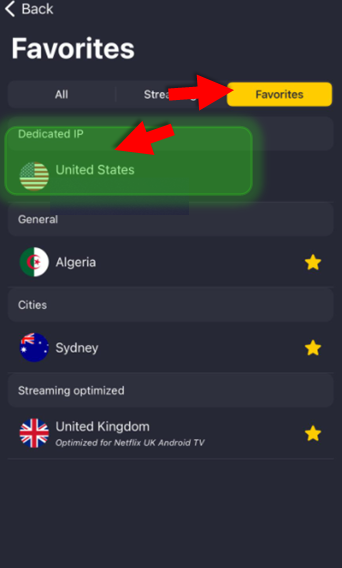The image is a screenshot taken from a mobile device showcasing various elements of an app interface against a dark gray background. In the upper left corner, there is a white "Back" button with a leftward-pointing arrow. Directly below it, the word "Favorites" is written in white text. Adjacent to this is a yellow favorites bar, highlighted by a large red arrow pointing right towards it.

Further down, a green bar labeled "Dedicated IP" features an American flag and is marked by another red arrow, this time pointing left towards the flag. Below the green bar, the word "General" appears in white text, accompanied by the flag of Algeria. Next, the label "Cities" is written in white, positioned above an Australian flag with the word "Sydney" next to it.